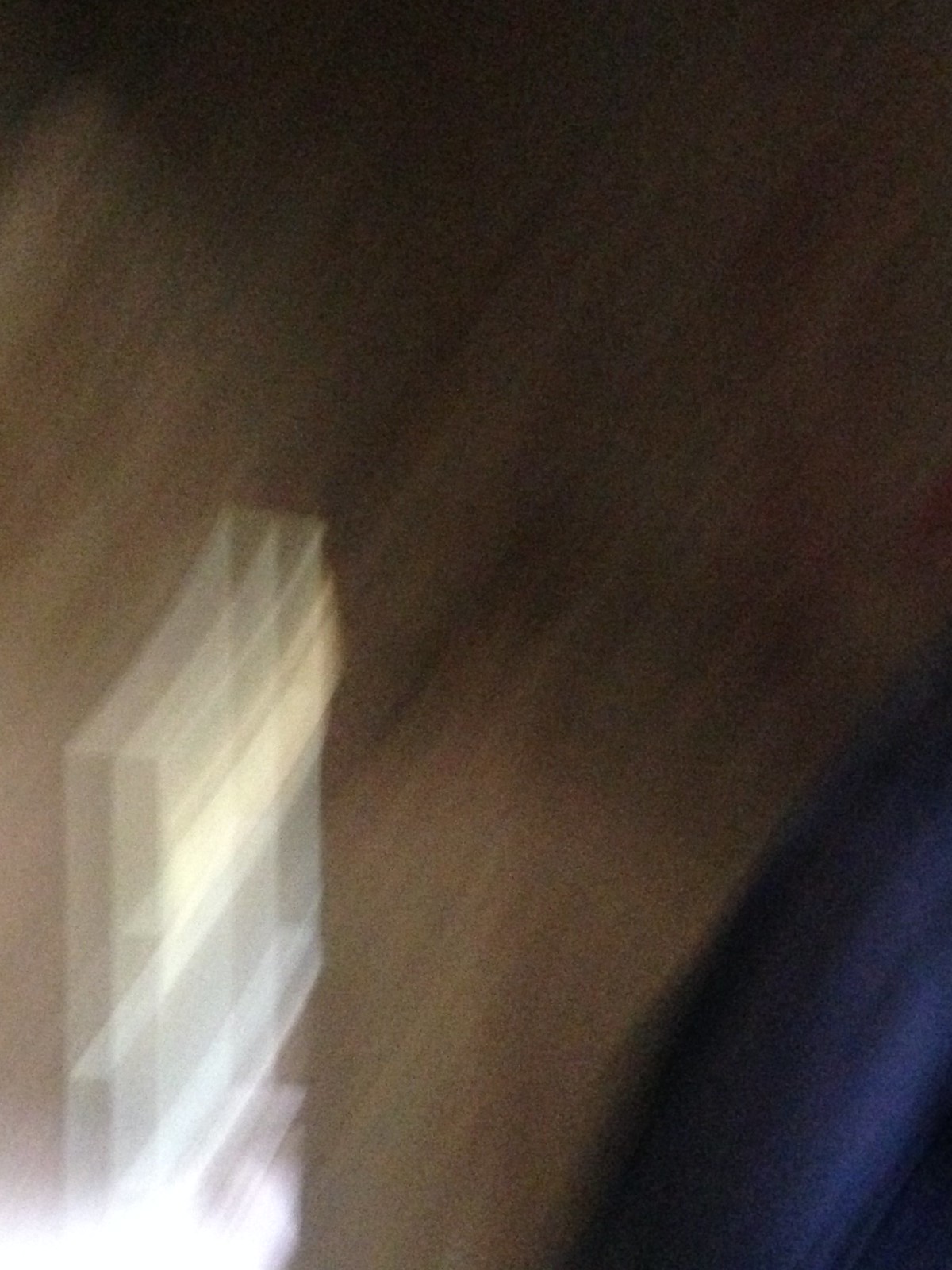This photograph is extremely blurry, making it challenging to identify clear details, but certain elements can be described. The image features a mix of colors, predominantly browns, yellows, whites, and blues. The bottom left-hand corner is dominated by a bright white light that blurs out part of the image. There appear to be three straight lines of white and yellow, creating a tripled effect with shadowed boxes. The bottom right corner is a smear of navy blue, transitioning to black towards the top right corner. The center and majority of the image show a brown color, possibly indicating a wooden surface or wall. Some suggest that it may depict a brown paneled wall with plastic containers used for holding papers or file folders, commonly found in offices. The overall composition is further characterized by lines that are somewhat diagonal, adding to the perception of motion blur. Additionally, there might be an indication of a window with intersecting vertical and horizontal lines, contributing to the abstract and indistinct nature of the photograph.